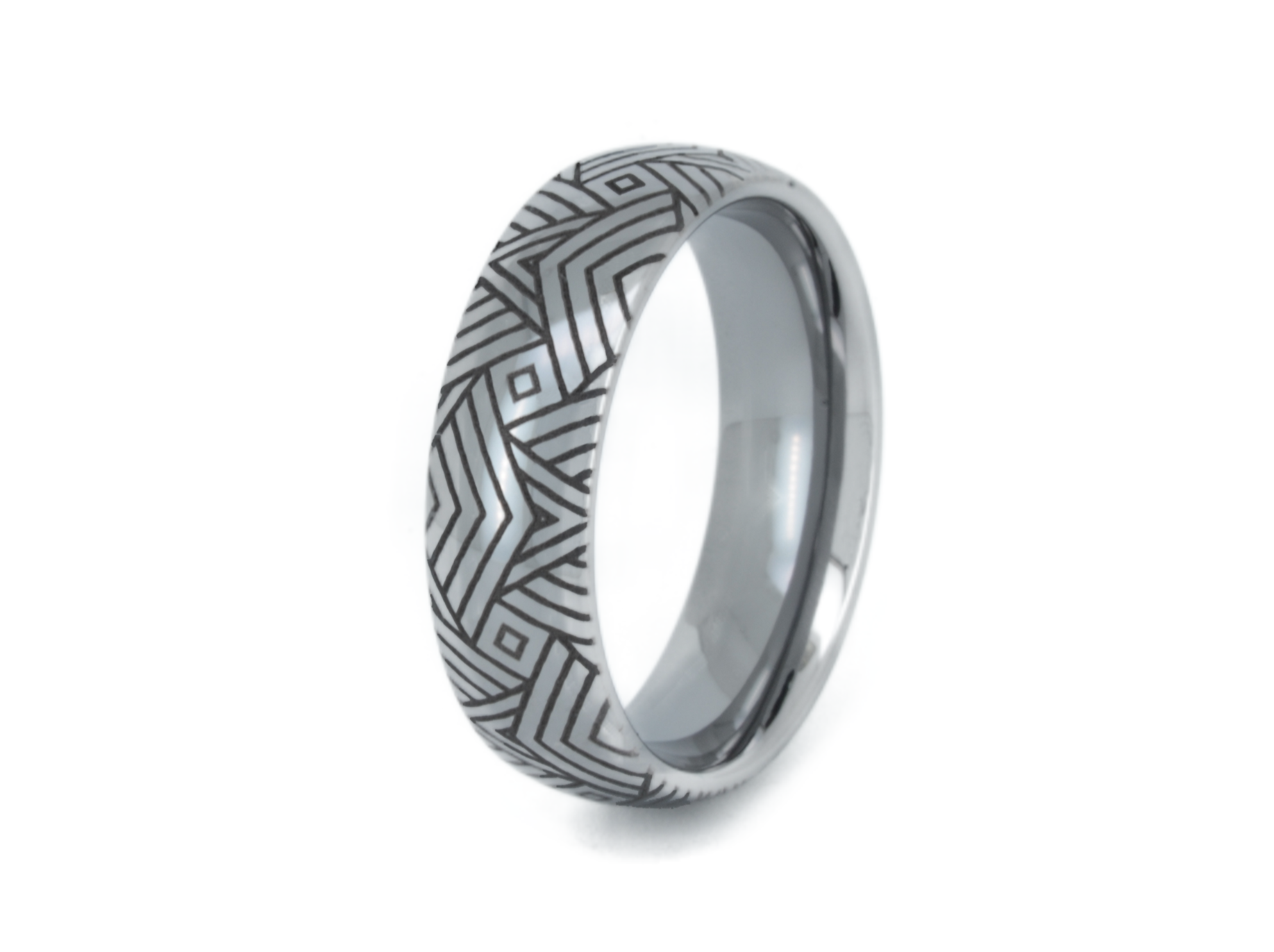This image features a silver ring positioned upright against a solid white background, highlighting its intricate design. The ring, likely made of titanium, brushed aluminum, or stainless steel, is sized appropriately for a typical human finger. It boasts a smooth concave inner surface. The outer surface is adorned with a distinctive pattern of black lines that intermingle, forming various geometric shapes such as squares, diamonds, triangles, and boomerang-like patterns. These black lines create a visually striking, almost trippy design, enhancing the ring's otherwise simple silver appearance.